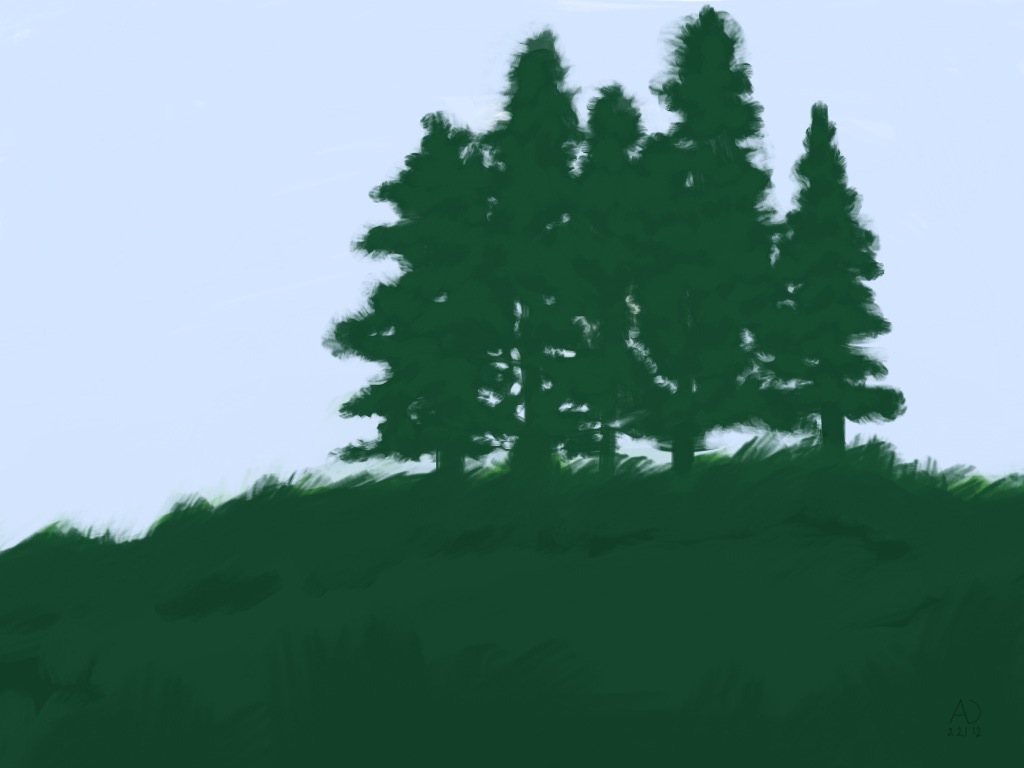A cluster of five vibrant green trees stands together atop a hill, with lush grass of a matching shade sprawling below. The scene has an animated or perhaps painted quality, with the grass and trees both exhibiting a texture resembling soft, fluffy animal hair. Multiple shades of green are used to create a sense of depth through shadows. The backdrop is a clear blue sky, adding a serene contrast to the rich greenery of the landscape.